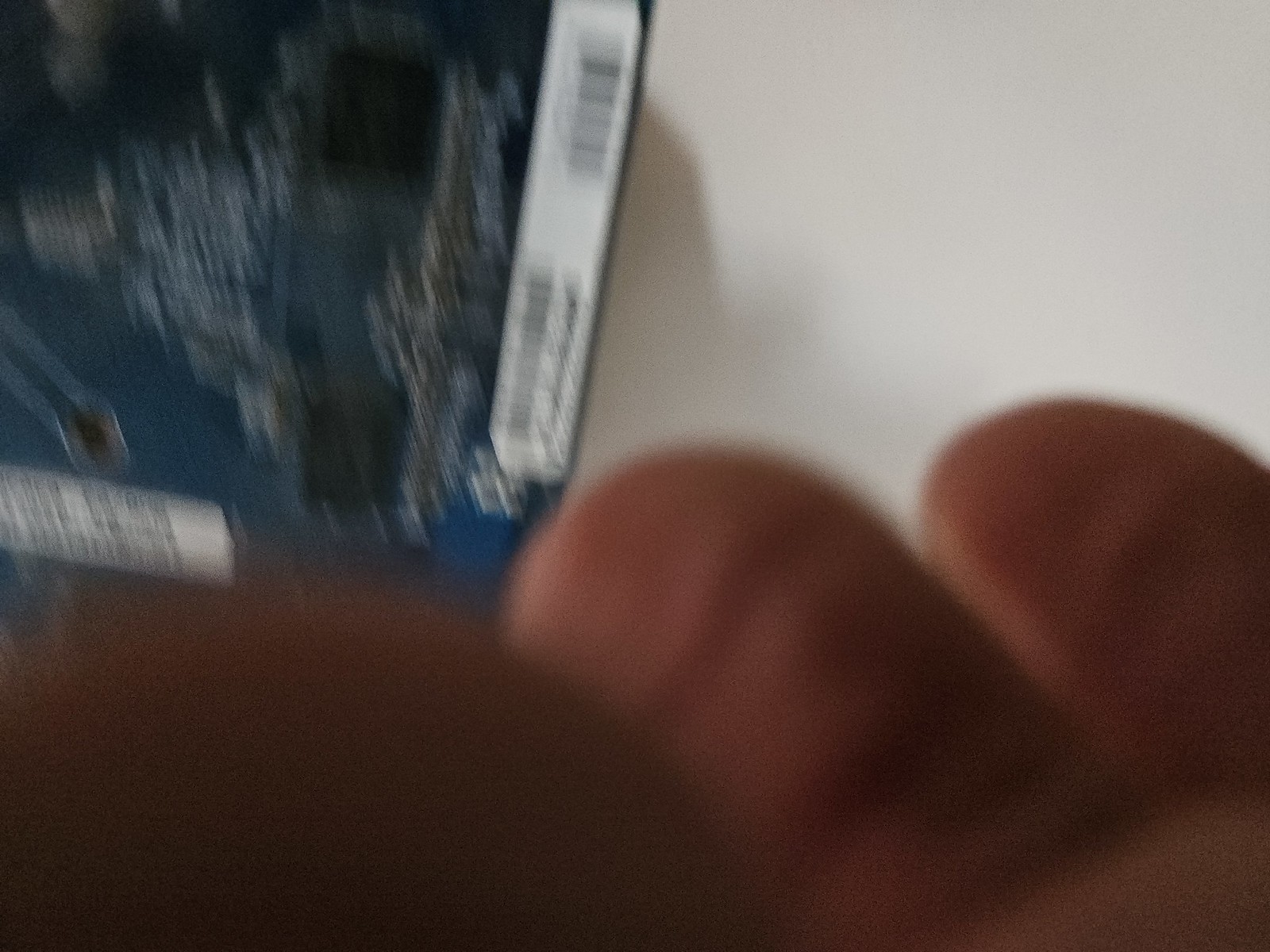This image captures a blurred scene that makes identifying specific elements challenging. Predominantly occupying the bottom third of the frame are what appear to be three appendages, likely toes, given their light skin tone and distinct nubs. The ambient light casts faint shadows that add to the indistinct appearance of these toes. Beyond them, a white wall forms the background, creating a stark contrast. In the image's top left corner, there is a partially visible poster or artwork. This poster features a predominantly blue design, interspersed with white boxes that contain barcodes, though the motion blur obscures any finer details. The overall effect is one of dynamic movement, leaving the viewer with a sense of curiosity about the scene's true nature.